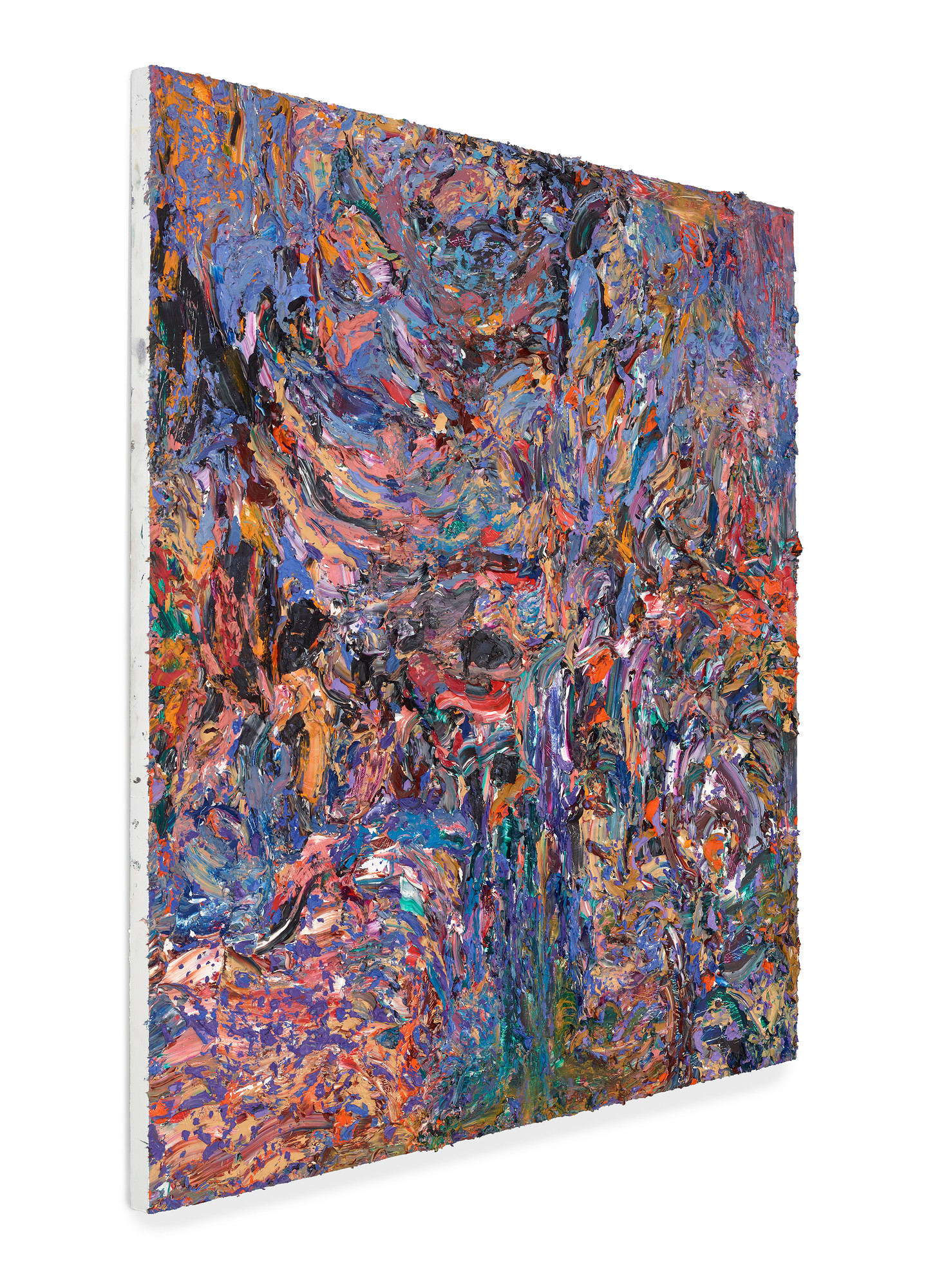The image showcases an abstract painting on a rectangular canvas with a plain white background. The painting is slightly rotated, presenting a three-dimensional view where the left edge of the canvas appears closer and higher (approximately four to five inches) than the right edge (around three to four inches high). The canvas itself is taller than it is wide, with an unpainted light gray edge on the left side, showing hints of paint smudges. This avant-garde painting utilizes layers of acrylic paint to build texture, featuring a chaotic blend of vibrant colors such as various shades of blue, purple, orange, red, bright and dark orange, black, brown, gray, yellow, white, and occasional hints of green. All the colors appear to be applied with no particular direction, creating a dense and dynamic amalgamation that lacks any discernible shapes or patterns, offering a raw and unstructured visual experience. The center of the painting features a slight concentration of red hues amidst the chaotic display.